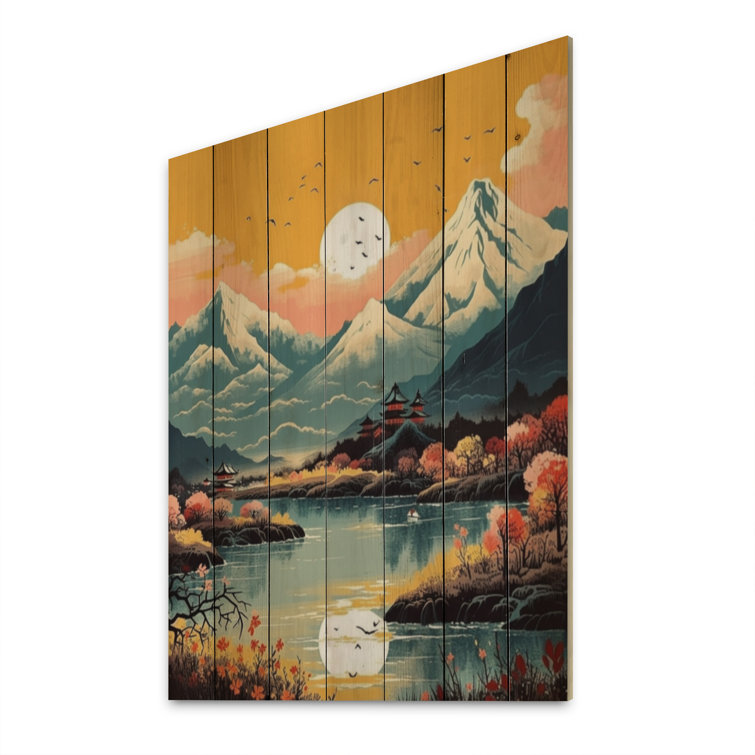This artist's captivating painting is rendered on six vertical brown wooden planks, creating an intricately detailed Asian landscape. The piece spans approximately six feet tall by five feet wide and is rich with vibrant colors and natural elements. Starting at the top, an orange sky features either a moon or sun, with birds flying in silhouette against pink clouds. Below this celestial scene, snowy blue mountains rise prominently, growing darker as they approach the foreground. Nestled near the base of the mountains is a traditional Japanese temple, painted in striking hues of red, black, and blue. Further down, the landscape bursts into the vivid colors of fall with bushes and trees in shades of yellow, pink, red, and green cherry blossoms. Flowing through the middle, a blue river captures the reflection of the distant mountains and the celestial body above, adding a touch of serene beauty to this exquisite work of art.